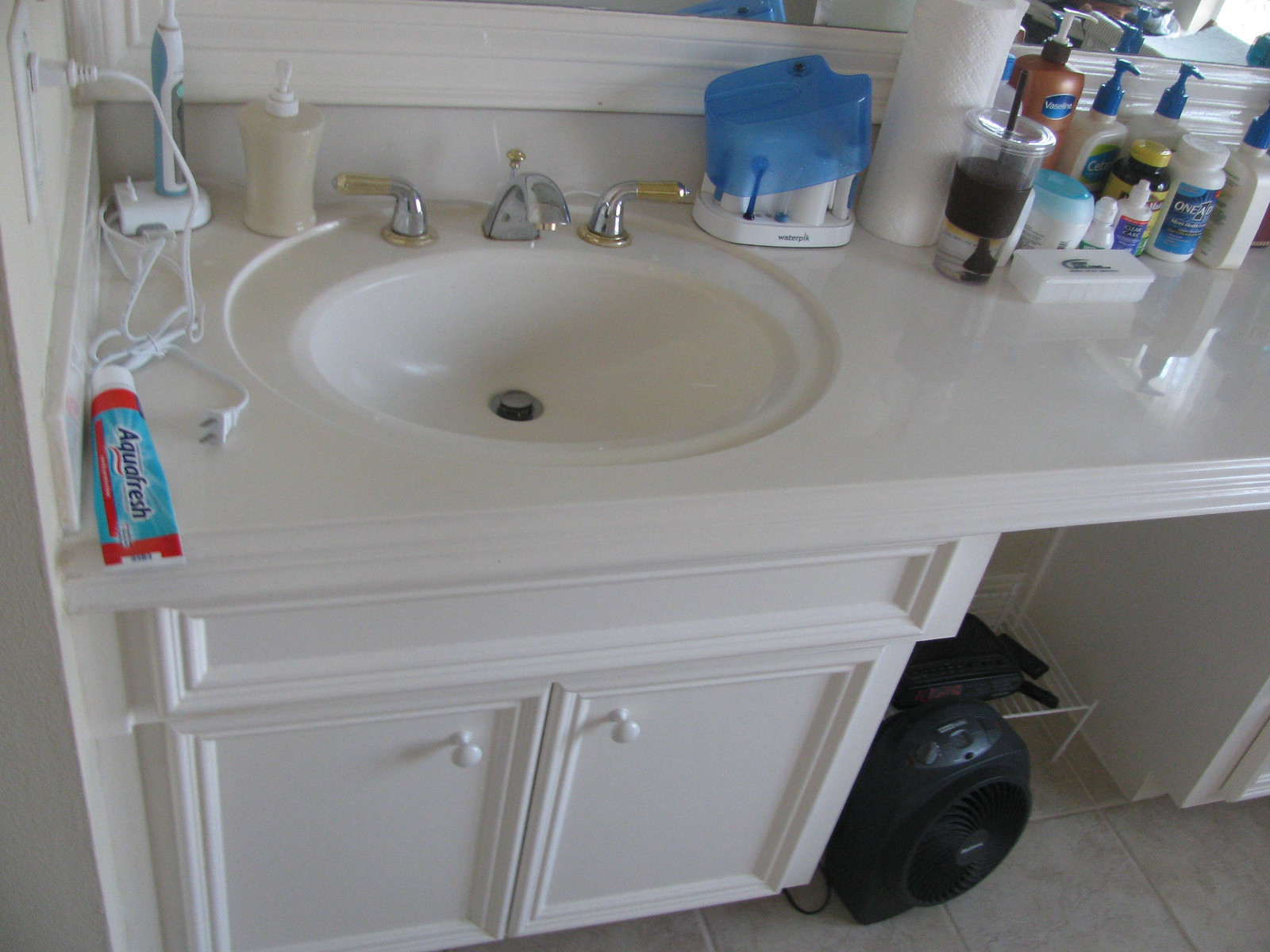The image features a detailed view of a bathroom countertop and sink area. On the far left, a section of the white wall is visible, with an electrical outlet in the upper left corner. From this outlet, a white cord descends, connecting to a blue and purple electric toothbrush situated at the upper left corner of the counter.

Next to the electric toothbrush is a beige-colored soap bottle equipped with a squirt top. The countertop, which appears to be white with subtle flecks, supports an under-mounted basin also in white. The sink is flanked by a silver faucet, with gold accents on the tips of the handles and around the base of the handles. The sink features a matching silver-and-gold drain control plunger. 

To the right of the sink sits a dental device resembling an ice pick with various heads, positioned in a clear holder. In front of this, closer to the left, is a tube of Aquafresh toothpaste. The toothpaste has a blue body with dark blue "Aquafresh" text on a light blue background, highlighted by red stripes on the top and bottom. The white cap is oriented towards the back of the counter.

Below the countertop are two cabinet doors that open in the middle. Adjacent to this section is a black round heater or similar appliance, slightly recessed under the counter, accompanied by another dark-colored item.

A mirror extends above the sink, with its frame slightly visible towards the center-left of the image. Positioned close to the electric toothbrush and water pick, there is a tall, white cylindrical item. Next to this is a clear plastic cup with a black drink and a black straw.

The counter is further cluttered with various cosmetic items, including a long, white pillbox, eyedrops, powders, and creams with their corresponding dispensers. This assortment of personal care products is neatly arranged across the countertop, completing the detailed snapshot of this bathroom setting.